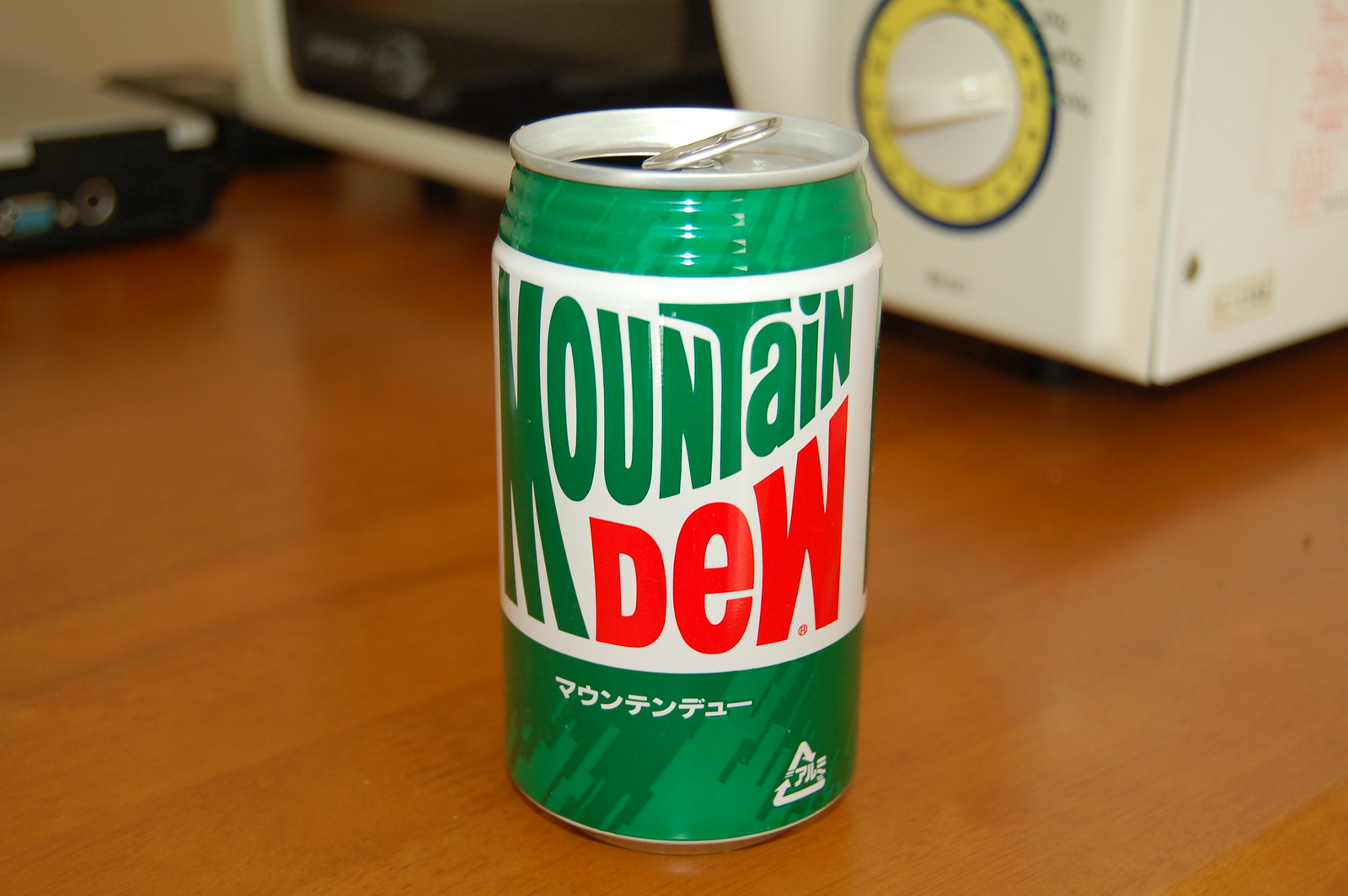A meticulously detailed photograph showcases a prominently positioned can of Mountain Dew, centered at the forefront. The brand name "Mountain Dew" is strikingly clear and legible, depicted in vibrant colors with "Mountain" in green and "Dew" in red. The can itself contrasts against a stark white background, framed by a vibrant green hue covering the remainder of the can. Importantly, the can is open, displaying that it has already been used.

Beneath the English branding, there are mysterious characters in what appears to be an Asian script, possibly Japanese, suggesting this might be a regional variant of the drink. These characters add an intriguing element of mystery, inviting curiosity about their meaning.

The can is stationed on a rustic brown wooden table, evoking a homely, comfortable atmosphere. In the background, partially visible, is a white microwave adorned with a distinctive circular blue and yellow dial, suggesting the setting is a kitchen. The placement of the objects suggests a casual, everyday scene, with the can likely being enjoyed as part of a regular kitchen routine.